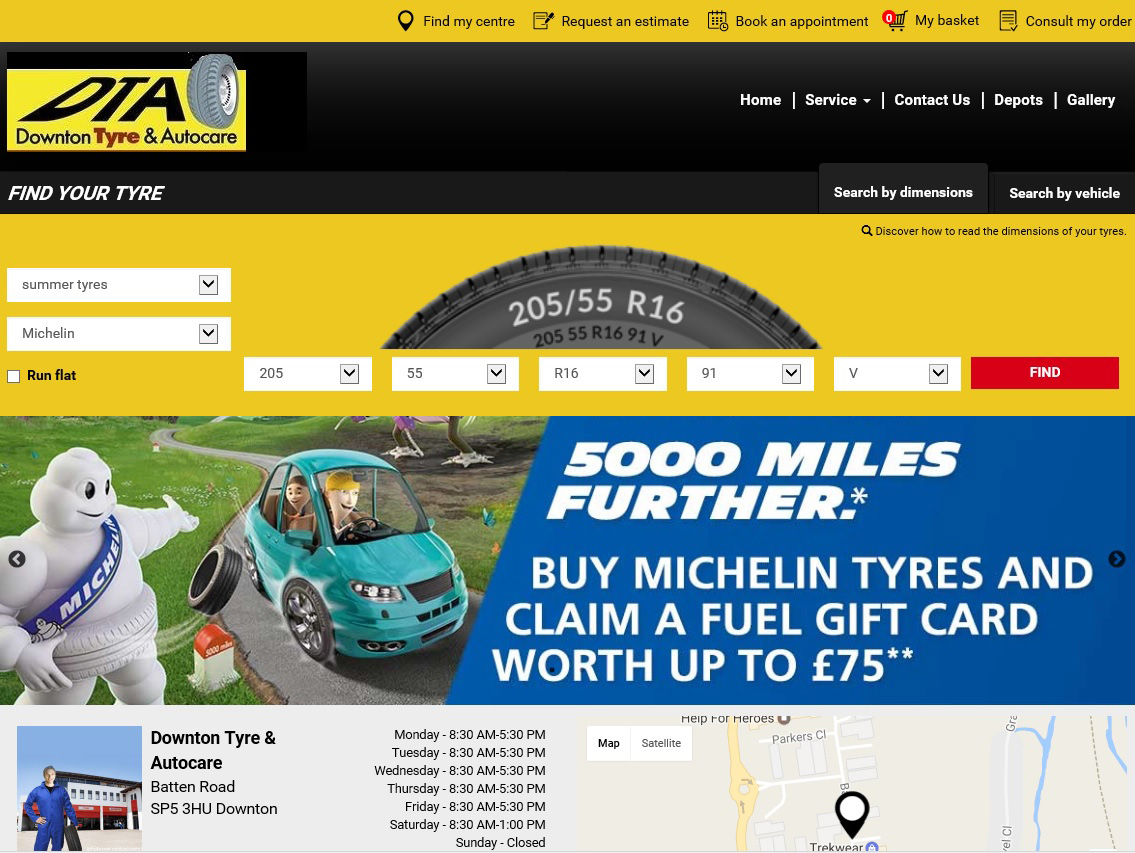This screenshot showcases a webpage primarily featuring a yellow background. Dominating the top section is a horizontal yellow rectangle. Just below this, a large black rectangle captures attention. In the upper left corner of the black rectangle, there is a smaller yellow rectangle with "DTA" prominently centered in big black letters. Adjacent to this is a standing gray tire displaying the rim and tread. Beneath this tire image, in black text, it reads “Downtown Tyre,” followed by “& Auto Care” in red.

To the right section, a white navigation menu lists: "Home," "Service," "Contact Us," "Depots," and "Gallery," each separated by vertical white lines. Immediately below, another line in white capital letters states, "FIND YOUR TYRE" on the left. On the right, there are two search bars captioned, "Search by Dimension" and "Search by Vehicle."

Further down, a horizontal yellow rectangle highlights a black tire with the inscription "2055/55 R16" in white on its outer edge. Beneath this, two additional search bars are positioned on the left side and horizontally across the bottom.

Continuing downward, a rectangle contains an image on the left featuring the white Michelin tire mascot along with a small blue-green car. The right side of this section, set against a blue background, proclaims “5,000 miles further.” Following this, there is an asterisk and a period. Below this slogan, it says, “Buy Michelin tyres and claim a fuel gift card worth up to £75,” ending with two asterisks. At the very bottom of the webpage is a map.